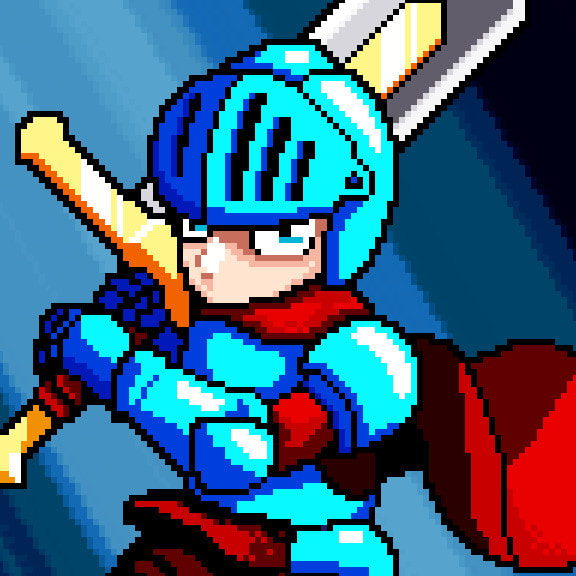This is a computer-animated, pixel art image depicting a knight in intricate, blue armor. The knight stands centered in the composition against a backdrop of diagonal blue stripes ranging from light to navy, with a black corner in the top right. His armor exhibits a striking contrast with the left half in teal and the right half in a deeper navy blue. He has pale blue eyes and is gazing to the left.

The character's ensemble features red accents around his arms and waist, and he's adorned with a flowing red cape that ties around his neck. The knight wields a large, impressive sword with a yellow handle and a blade of silver, highlighted by a blue section with a white outline and gold center. The image evokes a nostalgic retro vibe, reminiscent of graphic styles from the late 80s to early 90s.